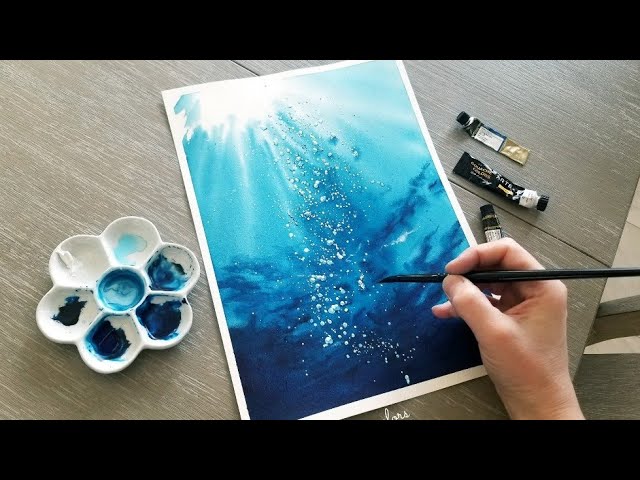This image shows a detailed scene of someone engrossed in creating a watercolor painting. The focus is on a white man's hand holding a very thin black paintbrush, dabbing dark blue paint onto a white sheet of paper set on a silver wooden design platform. The watercolor, which occupies the center of the table, portrays an underwater scene with various shades of blue, capturing the sunlight streaming through the water and forming bubbles amid the deep blue sea hue. 

To the left side of the table, which is light brown in color, rests a flower-shaped palette containing multiple shades of blue and some white paint, suggesting these were mixed to create different tints. On the right side of the image, three black paint tubes and a white plate are visible, adding to the artistic setup. This vivid depiction beautifully encapsulates the scene of creativity in process.